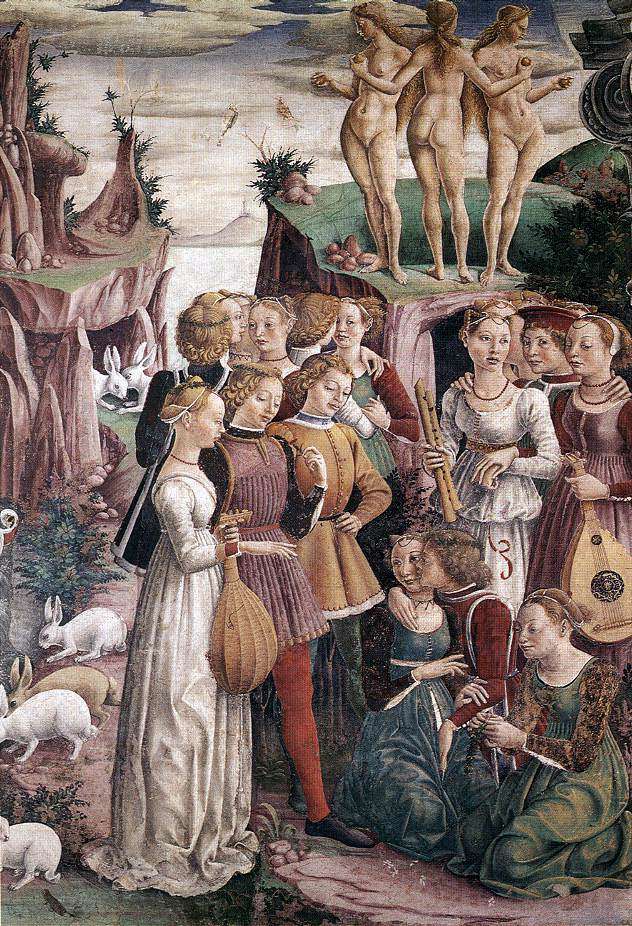This is a tall, intricate rectangular painting brimming with detail and characters, evocative of a 15th-century Bruegel piece. The background features a gradient sky that transitions from a grayish-blue to white near the horizon, punctuated by narrow dark gray clouds. To the left, a cliff formed of light pinkish rocks with light green surfaces stands, mirrored on the right side by another similar cliff. Atop the right cliff, three nude women with long, curly blonde hair and pale skin hold fruits in their hands. The central figure faces away while the two flanking her face forward, their heads slightly tilted downward.

In the middle ground below these cliffs, a group of predominantly female figures is gathered. They are dressed in elegant gowns and some in tunics with tights, presenting a scene of amorous interaction. One woman serenades with a lute, and another couple shares an intimate moment, suggesting a lively social gathering. Kneeling figures occupy the bottom right corner, adding to the richness of the scene.

To the left of this group and near the left cliff, several rabbits, both white and tan, are visible on the ground, adding a pastoral touch to the vivid, densely packed tableau.